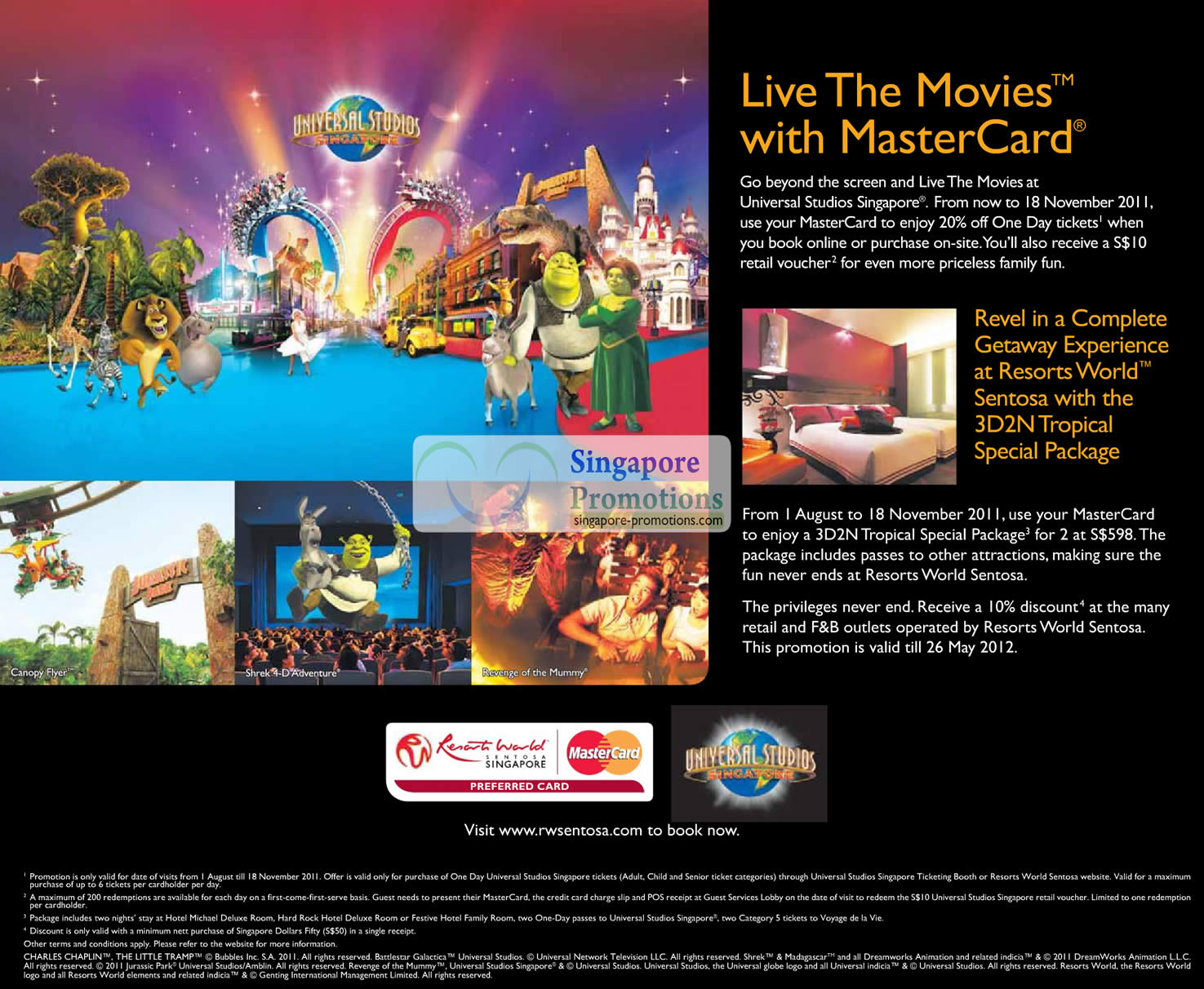**Universal Studios Singapore: An Unforgettable Movie Adventure**

Experience the magic of Universal Studios with this vibrant, eye-catching advertisement showcasing the best of Universal Studios Singapore. Front and center, beloved characters like Shrek, Donkey, and the cast from Madagascar come to life amidst a backdrop of lush greenery, enchanting castles, and whimsical landscapes, creating a fantastical world straight out of the movies.

Three additional images highlight the unique attractions and experiences awaiting visitors. One showcases the thrilling Jurassic Park, another features Shrek in his iconic adventures, and the last depicts a lively audience engrossed in a captivating live show. Prominently displayed text invites you to "Live the Movies with MasterCard," encouraging visitors to immerse themselves in the cinematic wonders of Universal Studios Singapore. 

From now until November 18th, 2011, MasterCard holders can enjoy a 20% discount on one-day tickets, whether booking online or purchasing on-site. Additionally, a $10 retail voucher adds to the priceless family fun.

The promotion extends to Resorts World Sentosa, where visitors can revel in the Tropical Special Package, offering a lavish 3-day, 2-night getaway. The advertisement, adorned with vivid and appealing graphics, concludes with logos of Resort World Singapore, MasterCard, and Universal Studios, cementing the partnership that promises an unforgettable adventure.